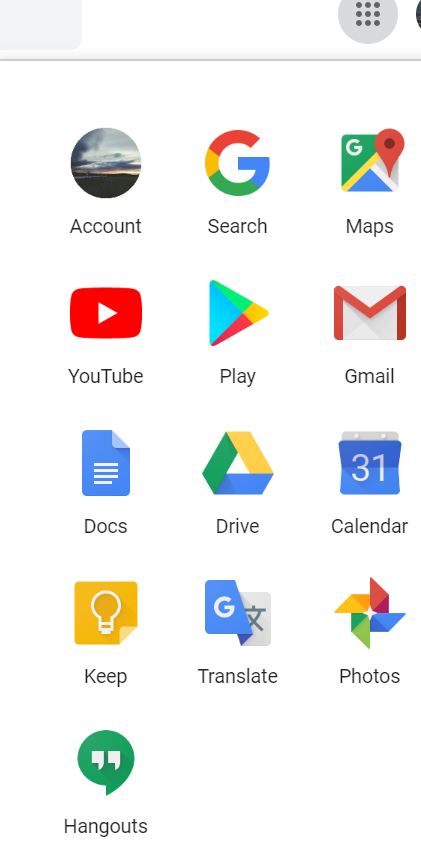A screenshot captures a mobile phone's home screen displaying a neatly organized collection of apps. At the top left, the first app icon displays a circular image labeled "Account," featuring a scenic picture that appears to be of an ocean view. Adjacent to it is the "Google Search" app, followed by "Google Maps."

The second row lines up with the "YouTube" app first, then the "Google Play" Store, and lastly, "Gmail." Continuing to the third row, the apps are "Google Docs," "Google Drive," and "Google Calendar." 

The fourth row begins with an app labeled "Keep," followed by "Google Translate" and "Google Photos." Concluding the series on the fifth and final row is the "Google Hangouts" app.

The overall arrangement highlights a strong preference for Google services, each app icon distinct and easily identifiable, making it evident that the user relies heavily on Google's ecosystem for their daily tasks and activities.